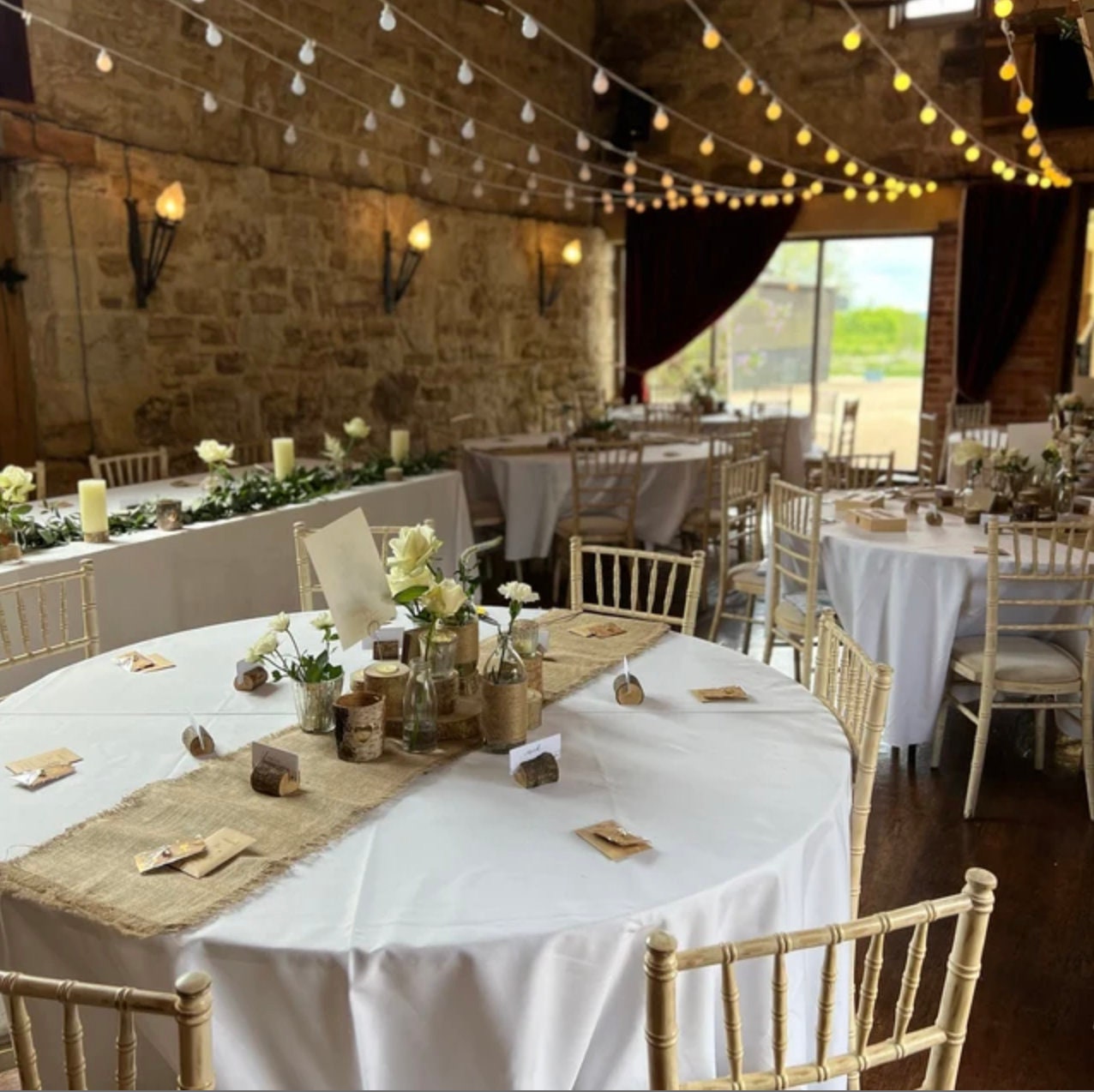This full-color vertically rectangular photograph captures the interior of a wedding reception hall illuminated by both artificial and natural light. The old masonry stone wall on the far left, composed of various sizes of bricks, adds a rustic charm to the scene. Three torch-like wall lamps are mounted on this stone wall. The ceiling, which mirrors the stone aesthetic, is adorned with hanging lights, some of which are lit while others remain off.

Centered at the back of the hall is a sliding glass door, partially covered by a curtain on the upper left-hand corner. Through this door, one can glimpse an outdoor patio area, another building, a hill, a mountain, and the sky, all adding depth to the scene.

The room is meticulously set up for an event, with several round and long rectangular tables arranged for guests. Each table is covered with cloths and features floral centerpieces, candles, napkins, and table runners, though no plates are present yet. The seating consists of white, bamboo-like chairs. Notably, the bride and groom's table, positioned towards the center left, is significantly longer than the round guest tables, making it a focal point in the arrangement.